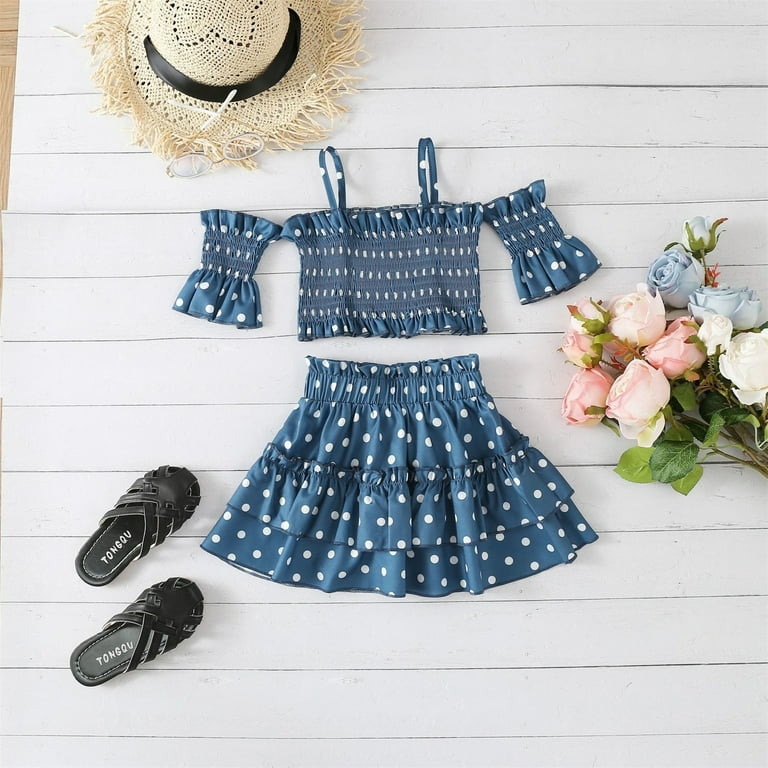The image is a portrait-oriented photograph showcasing a carefully arranged outfit for a young girl, laid out on a light blue, wooden deck or porch. Dominating the center is a charming blue dress featuring white polka dots on the sleeves and white diamond patterns on the bodice. The dress includes shoulder straps and open sleeves, with a waistband leading to a flared skirt with ruffles at the bottom. To the upper left of the dress, a tan straw sun hat with a black wraparound band is placed, adding a touch of summer flair. Close by, a pair of black crisscross leather sandals branded "Tongqu" rest on the deck, contributing a sense of small-scale fashion. Completing the scene, a vibrant bouquet of roses, comprising pink, blue, red, and yellow flowers with green leaves, lies to the right of the dress. The entire ensemble is set against the backdrop of the lined, light blue wooden surface, enhancing the charming and picturesque quality of the photograph.